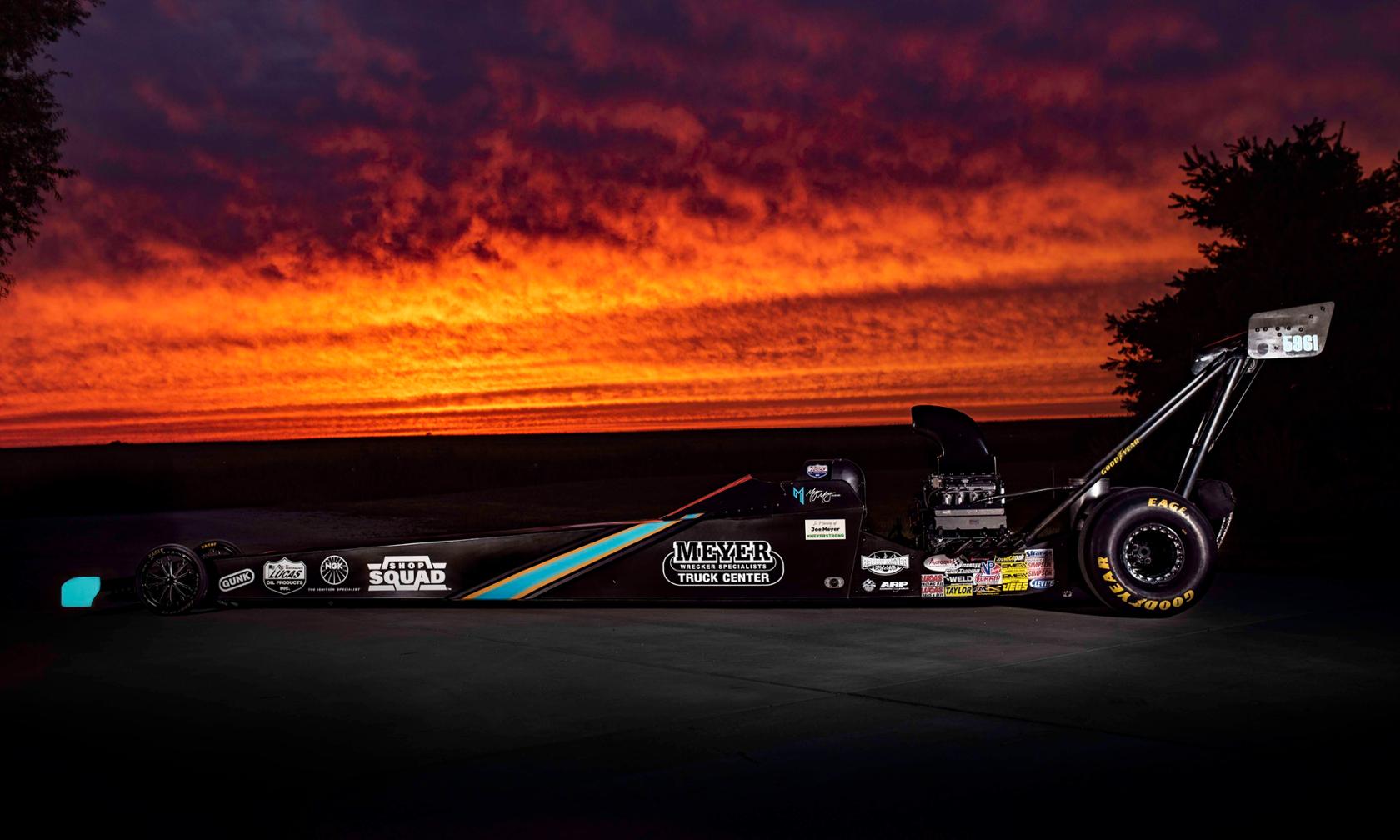This photograph captures an incredibly detailed and professional top fuel dragster at sunset. The black dragster, which looks almost triangular due to its design, features tiny, thin front tires and massive, wide rear tires. A tall, prominent wing (spoiler) dominates the back, while a large engine with an enormous scoop is positioned behind the cockpit. The car itself is elongated, with a narrow front section that comes to a point.

Logos, including "Meyer Truck Center" and multiple rectangular sponsor stickers, are displayed along the car's body, adding to its professional race-ready appearance. The dragster sits on a tarmac with a striking backdrop: a vibrant, almost surreal sunset sky. The brilliant red and gold hues of the sunset fade into a dark, almost black horizon, creating a stunning contrast. The clouds in the sky look almost like smoke, enhancing the dramatic atmosphere. A small blue bumper can be spotted at the front, and a tree is faintly visible in the background. The overall scene is one of both power and beauty, perfectly capturing the essence of a top fuel dragster in a high-quality photograph.